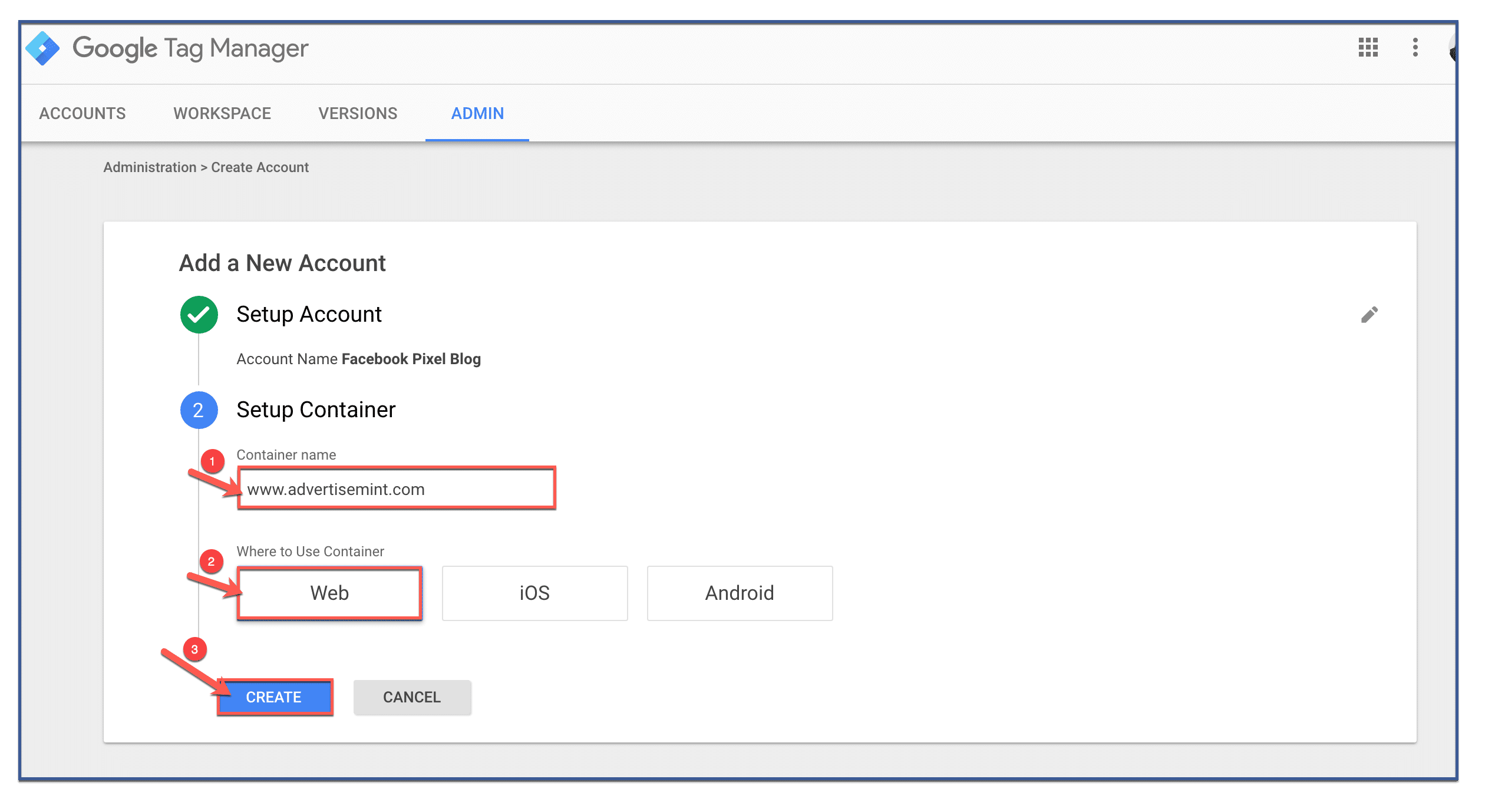This screenshot from Google Tag Manager showcases the "Admin" tab, which is highlighted in blue, indicating it is the active tab among the four available options: Accounts, Workspace, Versions, and Admin. 

Under the "Administration" section, the process of creating a new account is detailed. Step one, "Set Up Account," has been successfully completed, as indicated by a green checkmark. The account name given is "Facebook Pixel Blog." 

Step two, "Set Up Container," is currently in progress, shown in blue. The container name is specified as "www.advertisement.com" within the provided input box. Below the container name, the options for where to use the container—Web, iOS, and Android—are displayed.

At the bottom, there are two buttons: a blue "Create" button for proceeding and a gray "Cancel" button for aborting the process.

The screenshot has been annotated with red arrows and numbered steps that highlight the process. "Step 1" is marked with a red box around "Set Up Account," "Step 2" is indicated around "Set Up Container," and further instructions for "Container Name," "Where to Use Container," and the "Create" button are clearly marked for clarity.